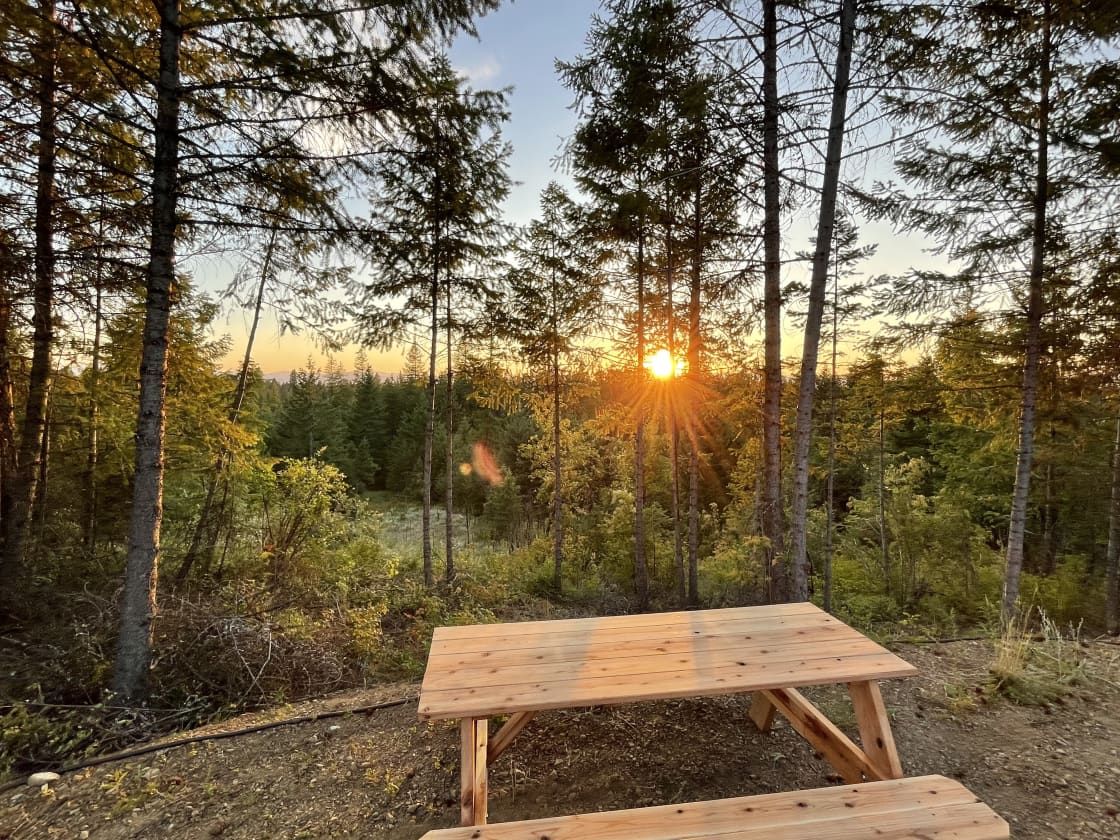In this vibrant photograph, a light-colored cedar picnic table with attached benches stands prominently in a well-kept dirt clearing, likely within a forest. Tall, slender trees frame the scene, their forms silhouetted against a sky transitioning from blue to the rich oranges and yellows of a setting sun. The sun’s rays cast a warm glow among the trees and illuminate the picnic table below. Stretching across the background, a black rope extends from left to right near the ground, with a distinctive white mushroom growing nearby. The setting exudes a serene, early evening ambiance, perfect for a peaceful moment amidst nature, accompanied by the sounds of birds and the promise of cicadas adding to the natural symphony.